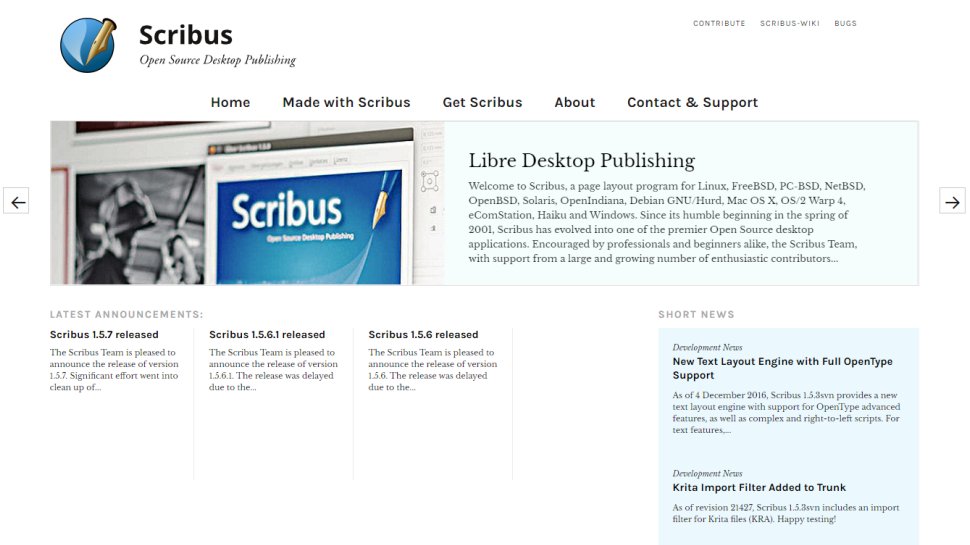Screenshot of a Scribbus webpage. The primary navigation bar at the top displays links to "Home," "Made with Scribbus," "Get Scribbus," "About," "Contact," and "Support." Below the navigation, an article features a discussion on desktop publishing accompanied by an image. Further down, three articles are listed under the heading "Latest Announcements." The highlighted article titled "Scribbus 1.5.7 Release" includes a prominent dark blue circular logo. The logo is segmented with a lighter blue section and features a pointed pen-like element indicative of writing or publishing.